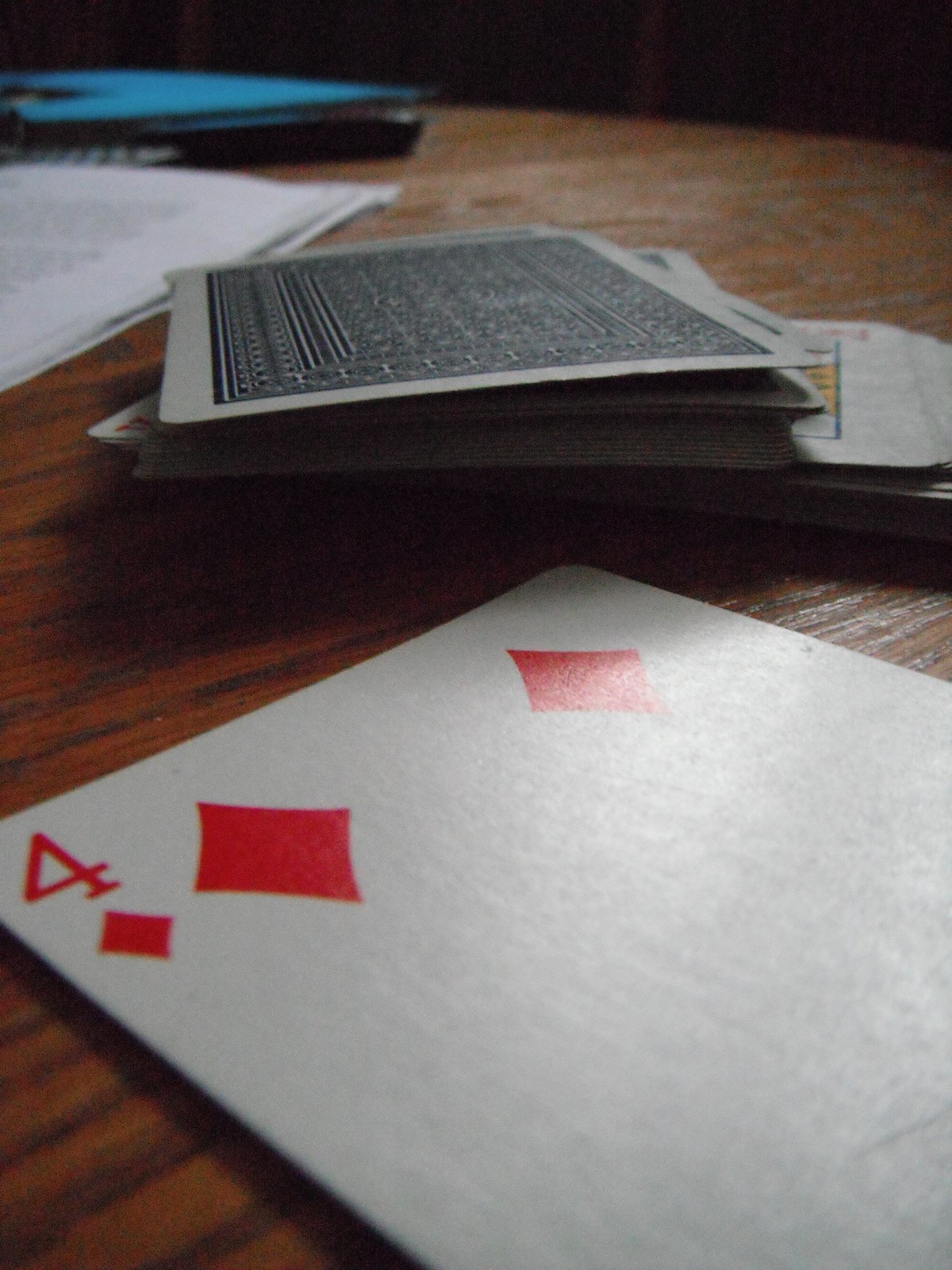This vertical color photograph features a detailed scene centered around a deck of cards. The focal point is the Four of Diamonds card, positioned diagonally and occupying almost the middle of the frame on the left side. This card appears prominently larger compared to the deck of cards situated in the lower right corner of the frame. The deck in the background is spread out in a somewhat haphazard manner, with both the faces and backs of the cards visible. One card face shows a red "K," indicating it's either the King of Hearts or the King of Diamonds.

The entire setup rests on a dark brown, varnished wooden table. The table's surface is accentuated with darker brown lines. Shadows from the disordered deck of cards fall onto the table, adding depth to the image.

In the upper left corner, a piece of paper with typed text is partially visible. Behind this paper, there is a long black and blue object that appears to be either a folder or a hole punch. The upper strip of the photograph is completely black, creating a stark contrast with the rest of the scene. This meticulously composed photograph captures the subtle details and textures of everyday objects, bringing an ordinary moment to vivid life.